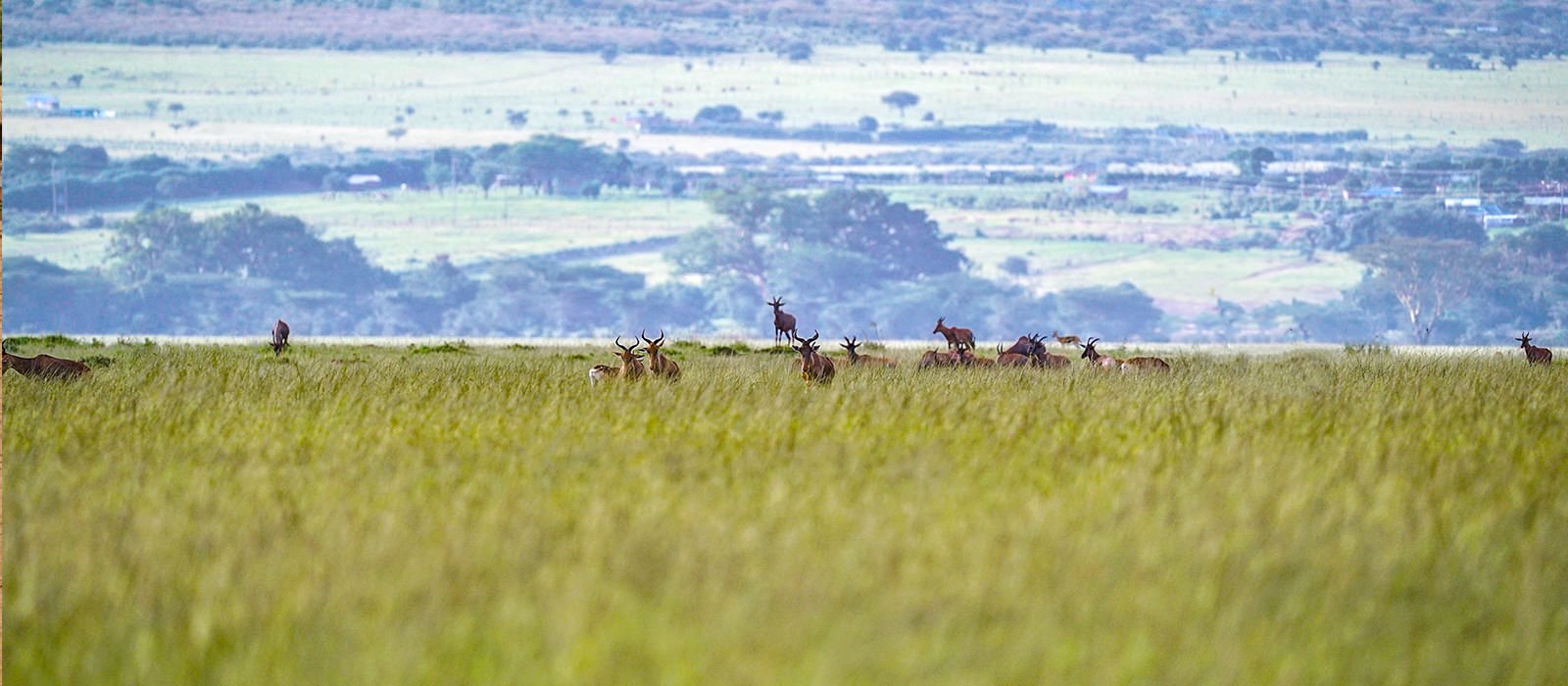In this photograph set outdoors, a group of approximately 13 antelope or gazelles are captured in a field of tall green grass. The photograph is taken from a distance, with much of the foreground blurred, drawing focus to the animals in the mid-ground. These brown, four-legged creatures, characterized by their thick bodies and distinctive curved horns, exhibit various postures: some stand, some rest on the ground, and one appears to be bending down to drink from an unseen water source. Beyond them, a serene body of water leads into a backdrop of trees and open countryside, extending into the horizon where the scenery blurs into a dreamy, faded image of an expansive African landscape. The natural beauty of the setting, potentially a large wildlife refuge, evokes the vast plains of Africa, suggesting a haven for these majestic creatures. No text appears in the image, allowing the focus to purely be on the tranquil and wild ambiance.